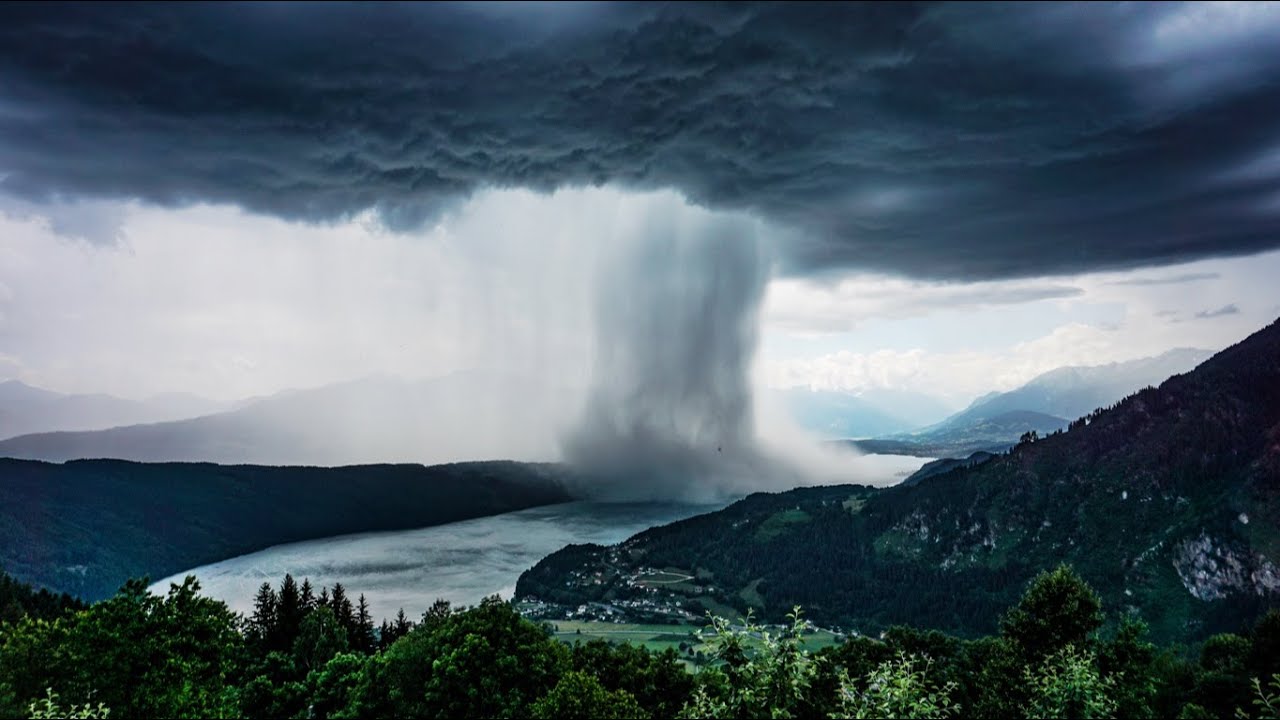The image depicts a dramatic, almost apocalyptic scene likely reminiscent of doomsday visuals from movies. Dominating the upper portion of the photograph is a massive, ominous dark blue and black-streaked cloud, giving the sky a foreboding appearance. A colossal plume of smoke or mist descends from this cloud to the ground below, obscuring much of the view and contributing to a pervasive haze throughout the scene. 

In the foreground, the tops of dark green trees interspersed with lighter green plants form a dense canopy, though their trunks remain hidden. The terrain features two lush, green hillsides, with the one on the right being noticeably larger and darker than the one on the left. A river, likely filled with grayish-blue water, snakes its way between these hills, adding to the surreal and eerie quality of the landscape. Behind the nearer hills, a more faded, distant hill is visible. The otherwise dark and brooding sky shows patches of white and lighter gray, particularly on the left side, which further emphasizes the turbulent atmosphere of the scene.